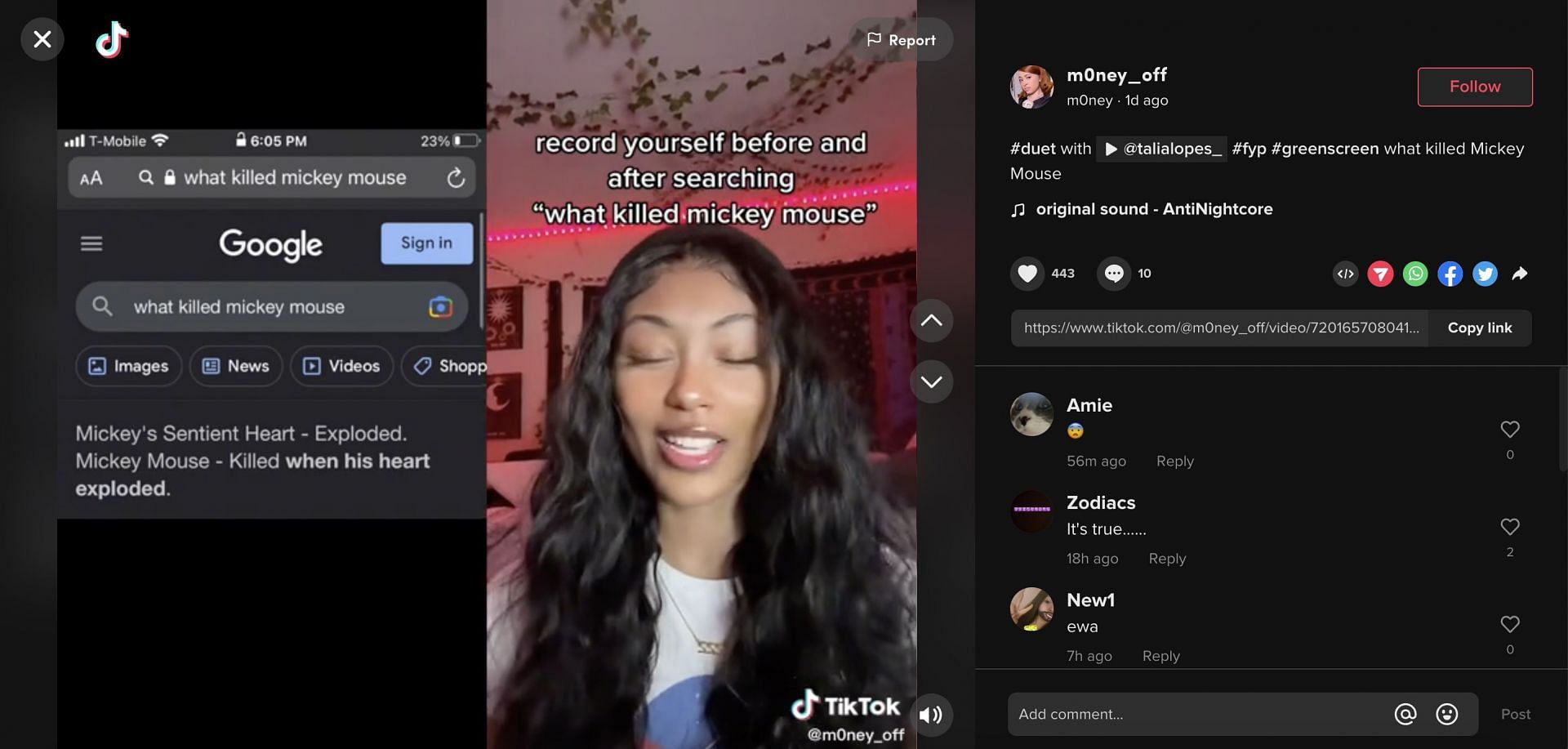This TikTok screenshot captures a poignant moment featuring a woman with long, wavy dark hair and dark skin, looking down with her eyes closed and mouth open. It appears to be a still shot from a TikTok video, where she participates in the trend: "Record yourself before and after searching 'What killed Mickey Mouse'." On the bottom right, the TikTok logo is prominently displayed alongside the handle '@m0ney_off'. To the left, a Google search query and results are shown, detailing that Mickey Mouse's sentient heart exploded. On the right, the interface shows various text overlays such as "money off", "#duet with @thalia_lopes_", "#fyp", "#greenscreen", "What killed Mickey Mouse", "follow", "original sound - anti-Nightcore", 443 likes, and 10 replies. Prominent comments include "Amy, the freaked out emoji, Zodiacs, replied, 'It's true.'" and "New one replied, 'EWA'." Additionally, a prompt to "add comment" is visible at the bottom of the screen.